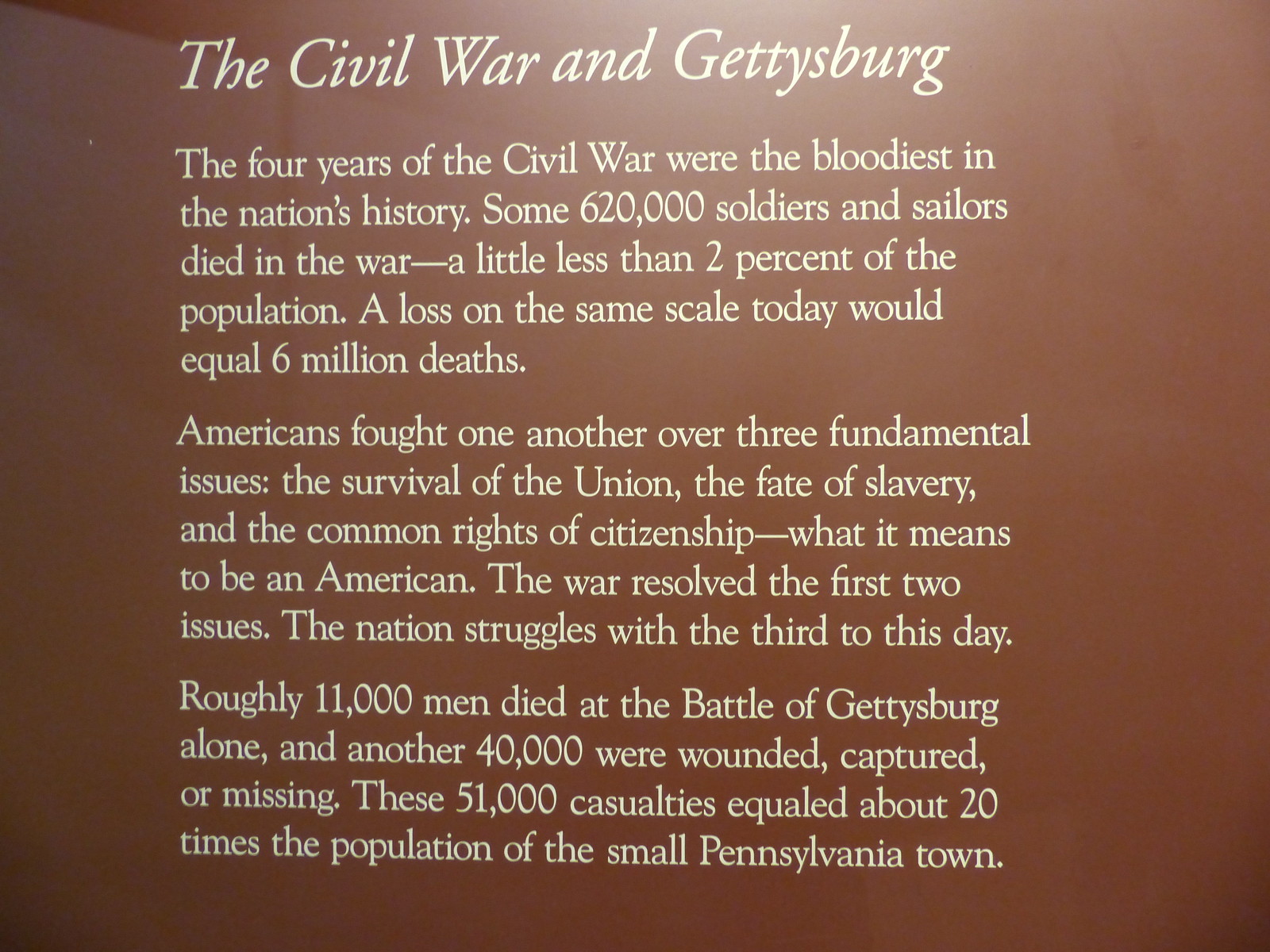This image depicts an informational card with a brown background and off-white or cream-colored text. The title at the top, written in italics, reads "The Civil War and Gettysburg." Below the title, in standard print, there are three paragraphs separated by spaces, which provide detailed historical information. The text explains that the American Civil War was the bloodiest conflict in the nation's history, resulting in approximately 620,000 soldier and sailor deaths, nearly 2% of the population at the time. If such a loss occurred today, it would equate to 6 million deaths. It highlights that Americans fought over three key issues: the survival of the Union, the fate of slavery, and the common rights of citizenship, focusing on what it means to be an American. Although the war resolved the first two issues, the document notes that the third remains a point of struggle. Additionally, it details the casualties of the Battle of Gettysburg, stating that roughly 11,000 men died and another 40,000 were wounded, captured, or went missing, which constituted about 20 times the population of the small Pennsylvania town. This card could be found in a museum or historical textbook.